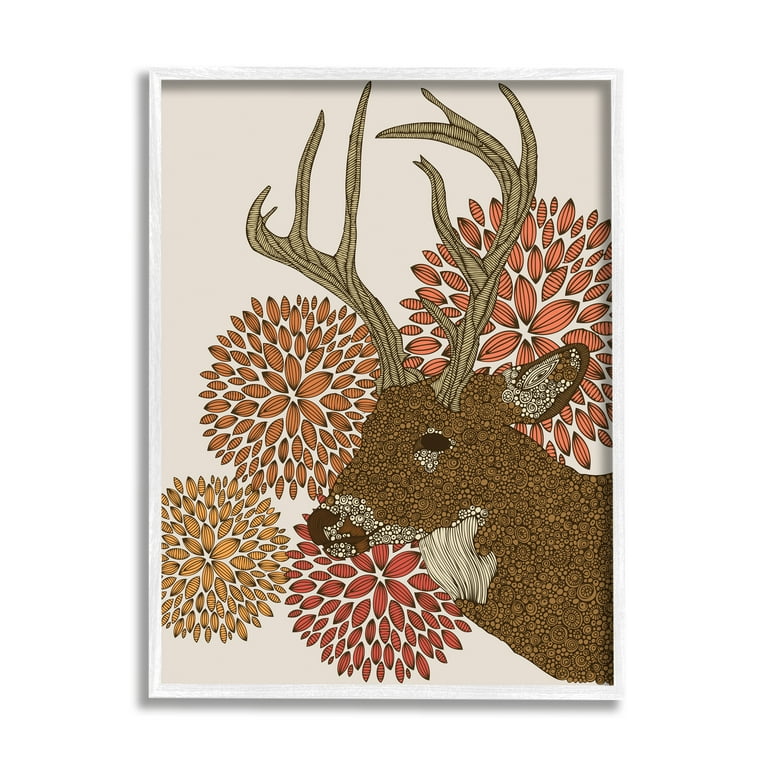This product photograph features a framed piece of computer-generated artwork, appearing to float against a stark white background. The rectangular frame, white and thin, highlights the central imagery—a detailed depiction of a deer, specifically a buck with tall, striped antlers. The deer's head is artistically rendered using various brown and tan swirl shapes, with white accents around its muzzle and neck. Surrounding the deer’s head are circular arrangements of four colorful, football-shaped flowers: vibrant orange, lighter orange, red, and yellow. This striking, abstract design seamlessly blends natural and geometric elements, creating a visually captivating and modern piece suitable for commercial use in online shops, listings, or catalogs.